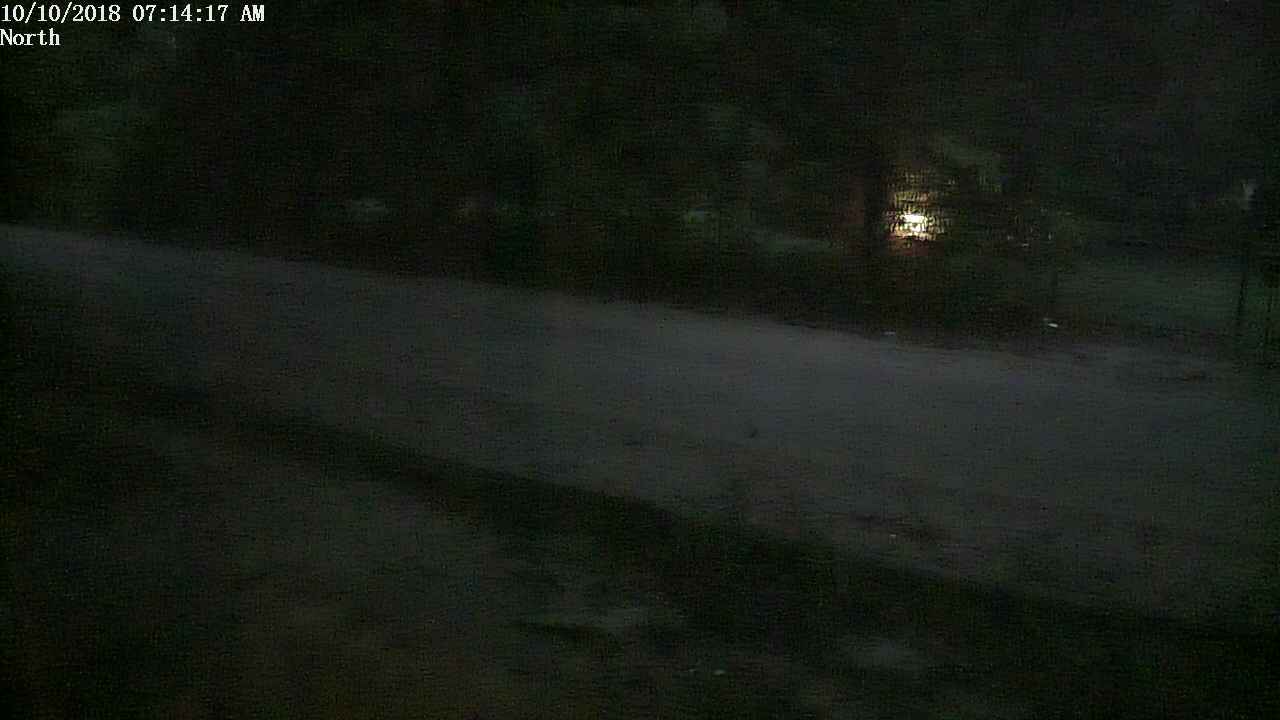A grainy, blurry, and dark nighttime image, likely captured by a security camera, shows a left-to-right rectangular scene. The poor texture and clarity make details hard to discern, but it appears to feature an outdoor setting. A muddy or wet road runs horizontally across the frame, lined by trees at the back. Towards the rear, a series of black fence posts connected by faint wires or chains are visible, with a grassy area behind them. In this grassy area, a yellow-white light or possibly a distant fire provides some illumination. In the bottom-left corner, there are hints of plants or a rocky area adjacent to the road. A timestamp and location data in the upper-left corner read "10/10/2018 07:14:17 AM NORTH," displayed in white letters.